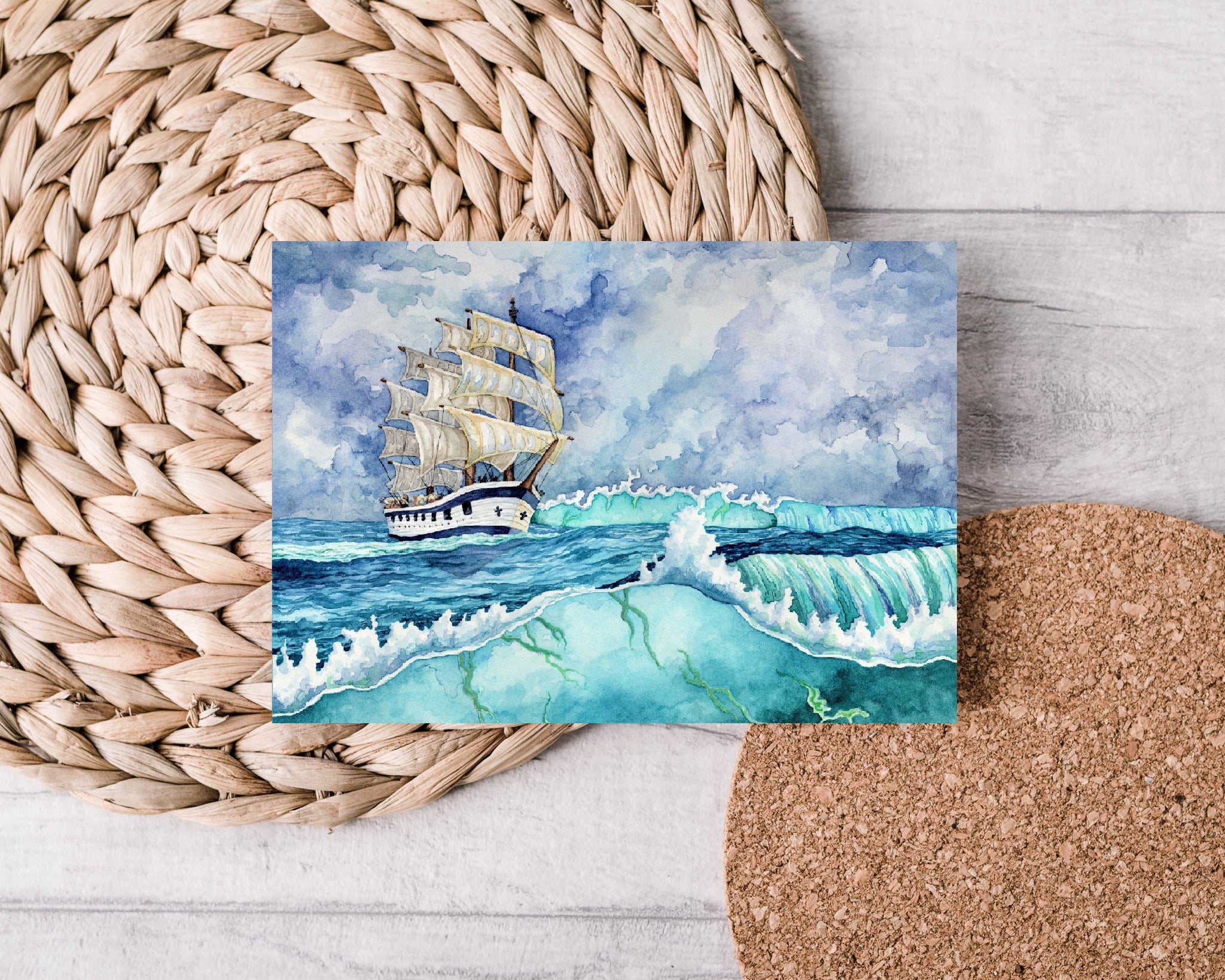This image features a small, square watercolor painting of an old-fashioned sailing ship navigating through turbulent waters. The ship, characterized by its three rows of long sails and a white hull with black stripes covering the cannon holes, cuts through blue and green waves under an overcast, bluish-dark sky. The painting rests on a wooden table, supported by distinct mats: a dense corkboard mat on the lower right and a braided, basket-weave mat on the upper left. The intricate mats, combined with the natural wooden texture of the table, provide a rustic backdrop that contrasts subtly with the mostly blue and green hues of the painting. The light source from the left casts a gentle illumination over the scene, enhancing the details of both the artwork and its unique setting.